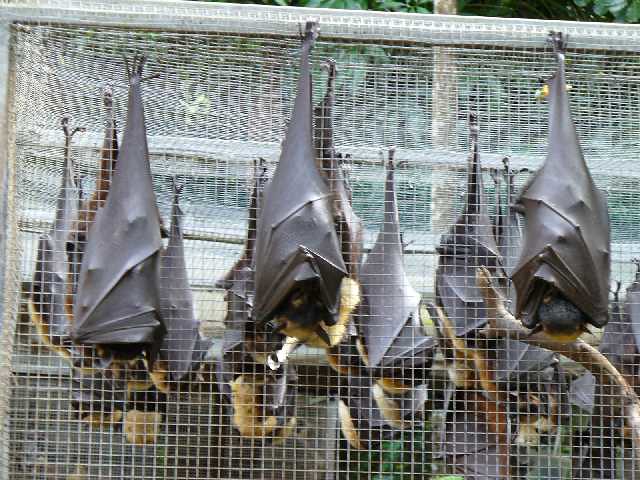The image shows a group of large, fruit bat-like creatures sleeping upside down, nestled within their giant, cocooned wings. They are attached to a white, netted structure that resembles a zoo enclosure with squares of narrow mesh. Among the bats, three are particularly visible on the front fence, revealing their little heads and gripping feet. Behind them, the blurred view shows at least seven more bats hanging inside this white net area, surrounded by some sticks or branches. The bats exhibit brown to black fur with hints of yellow, and their wings have a grayish-silver tinge. The backdrop includes trees and leaves, enhancing the enclosure's natural appearance, as the bats rest during the daytime.